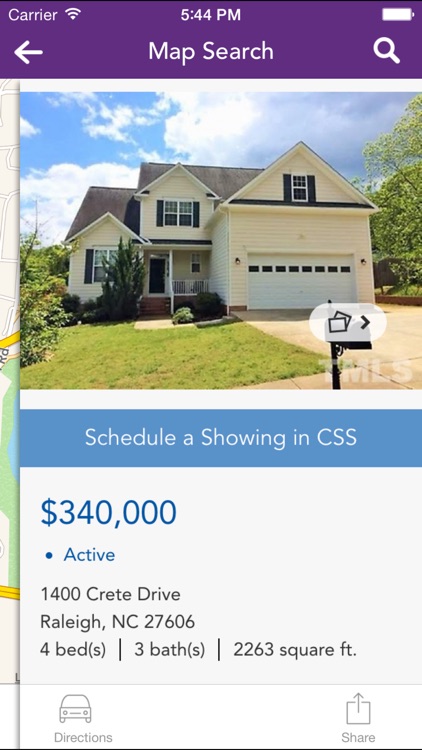This screenshot, taken from a smartphone, features a housing app. The phone's status bar displays a fully charged battery icon at the top right, the word "carrier" at the top left, and the time "5:44 PM" at the center top. 

The main content of the screenshot pertains to a real estate listing, likely for either renting or buying purposes. At the top of the app interface, the term "Map Search" is visible, indicating an option to view the property's location on a map.

Beneath this is an image of a cream-colored, two-story house with an additional attic space above a spacious garage. The garage appears wide enough to accommodate two regular-sized cars, with a window situated above it, signaling the presence of the attic.

Further details about the listing include an option to schedule a showing through "CSS." The property is listed at $340,000 and its status is marked as "Active." Additional information reveals that the house is located at a specific address (not fully provided in the screenshot) and includes four bedrooms, three bathrooms, and a total living space of 2,263 square feet.